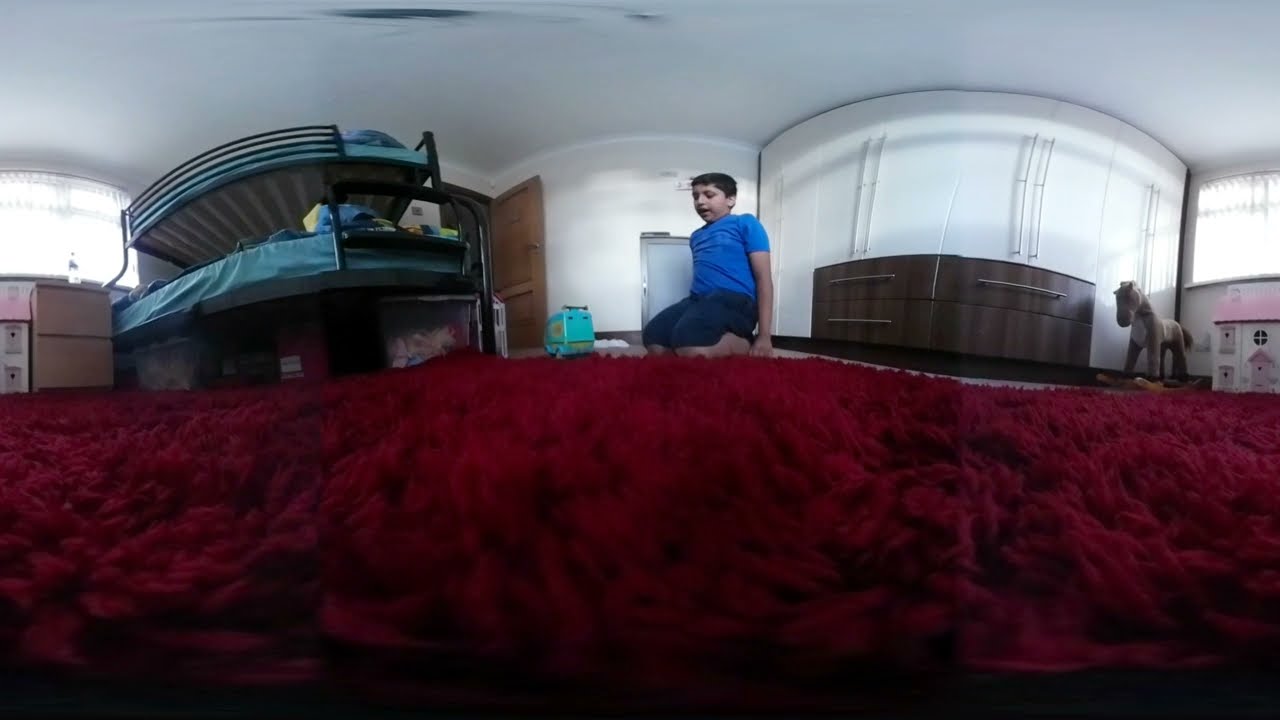The image is a fisheye or 360-degree view of a young boy, around seven years old, playing with a turquoise toy truck that resembles the Mystery Machine from Scooby-Doo. The boy, who has dark hair, is wearing a dark blue t-shirt and dark pants and is crouched on a red shag carpet that takes up the bottom half of the image. The room is painted white with bright light streaming through windows in the background. To the boy's left, there is a curved bunk bed with light blue sheets and railings, along with a box that likely contains toys. On the left side, there is also a small brown dresser with horizontal metal handles, missing one drawer pull, and a water bottle on top of it. To the right, there's a brown rocking horse next to a dollhouse with a pink roof and a wall comprising closet space or shelves.